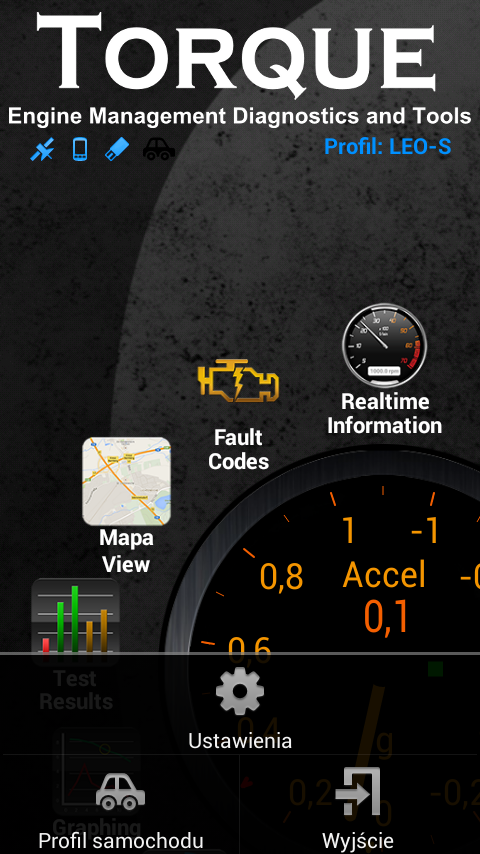The image portrays a user interface of a mobile application focused on automotive diagnostics and management. 

At the bottom of the screen, there are several clearly distinguishable icons resembling common app navigation tools, such as the settings icon, a car logo, and an exit door symbol likely for logging out or exiting the application.

The top section prominently displays the words "Torque, Engine Management, Diagnostics and Tools," indicating the app's primary functionalities.

In the middle portion, several sections and icons are visible. The central feature is an image of a car's dashboard, specifically highlighting a speedometer. Above the speedometer, the text "Real-time Information" is seen, next to a speedometer logo. Adjacent to this, there's an icon resembling a battery along with the label "Fault Codes."

To the left of this, a map icon is present, labeled "Map View." Below that, a bar chart icon is labeled "Test Results," implying a section for diagnostic test outcomes.

This detailed layout suggests a comprehensive tool for vehicle diagnostics and real-time monitoring, providing a variety of information and settings options to the user.